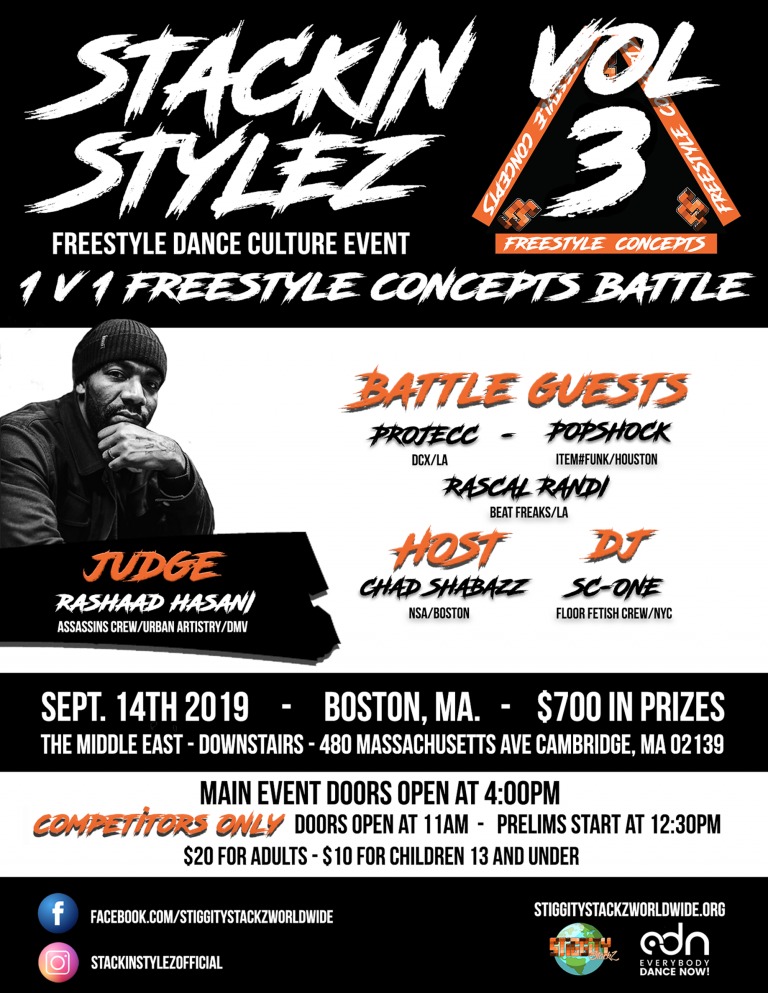This vertically aligned rectangular poster features various black and white sections. At the top is a black rectangular section with "Stackin Styles: Evolve 3" in bold white letters, followed by "Freestyle Dance Culture Event" and "1v1 Freestyle Concepts Battle." Below this, on a white background, there is a black and white photograph of a man with dark skin and a black beanie, resting his chin on his hand. The caption beneath the photo reads "JUDGE" in bold orange letters, followed by "Rashad Hassani" in bold white letters and affiliations: "Assassin's Crew / Urban Artistry / DMV."

To the right of the judge's information, "BATTLE GUESTS" is listed in bold orange letters with "ProTech - PopShock - Rascal Randy" underneath. Below this, details of the host and DJ are provided: "HOST Chad Shabazz" and "DJ SC1."

Further down, amidst two additional black rectangular sections, a white section prominently displays event details. It announces "MAIN EVENT," with doors opening at 4 p.m. for competitors only. Preliminary rounds begin at 12:30 p.m. with doors opening at 11 a.m. Ticket prices are $20 for adults and $10 for children aged 13 and under.